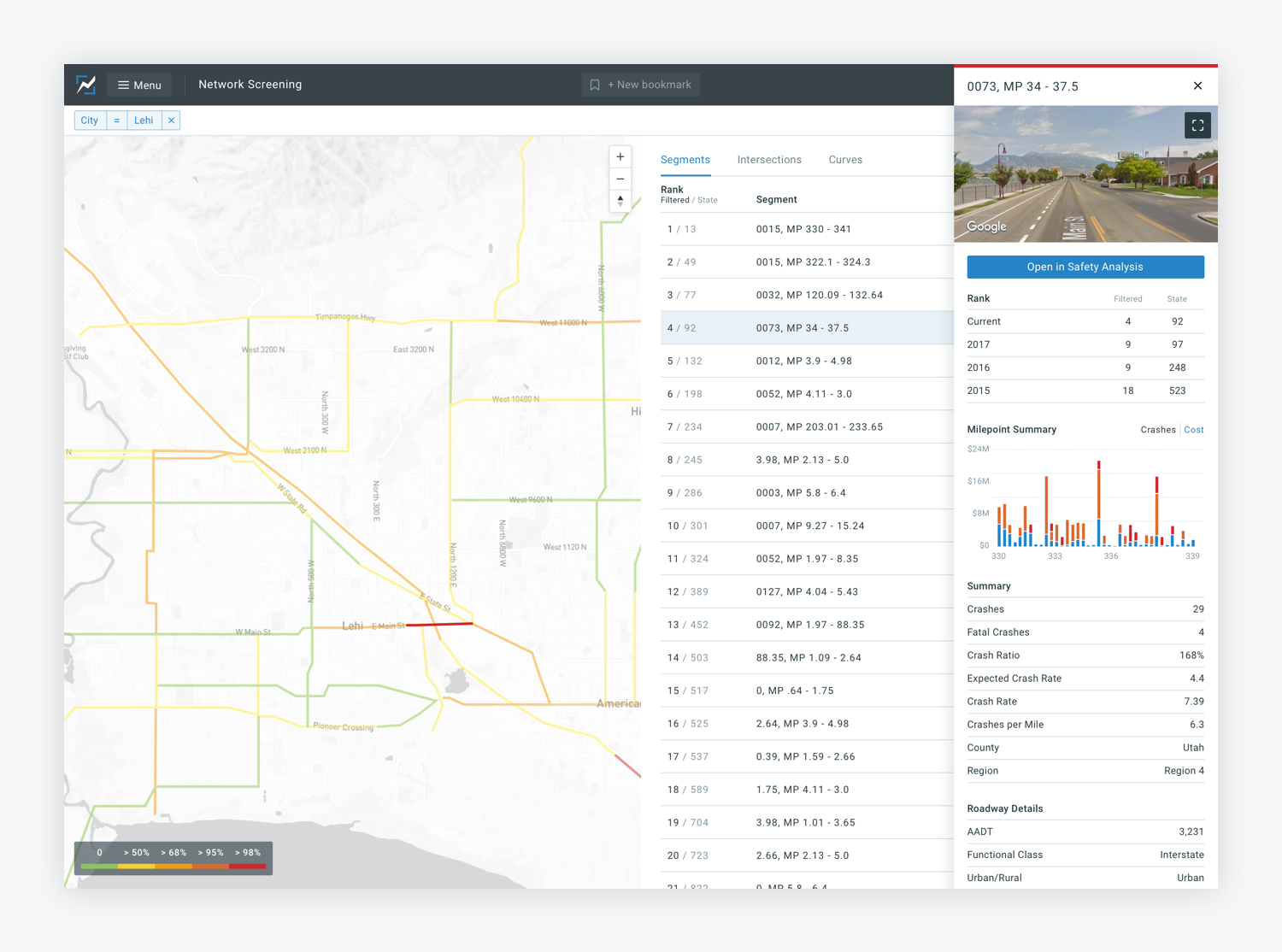The image displayed on the computer screen presents a complex and detailed visual interface. At the top of the screen, a horizontal black bar is prominently featured, displaying the labels "Menu" and "Network Screening." On the left side of the image, there is a map populated with various lines in different colors; these include yellow, light green, orange, and a small horizontal red line located about three-quarters down from the top and slightly to the right of the center. In the lower-left corner, a light gray key presents a color scale ranging from green to yellow to orange to darker orange, culminating in red, with corresponding numerical values above it.

To the right of the map, the screen is divided into two vertical columns. The first column lists the headings "Segments" (in turquoise), "Intersections" (in gray), and possibly "Curves" (the text is difficult to read) along with associated data that is too small to decipher, although we can discern columns labeled "Rank" and "Segment."

In the second column, at the top, a small horizontal red line is visible above an image of a roadway. This image shows a roadway lined with trees and a blue sky dotted with clouds. The road itself is marked with yellow and white lines. Directly beneath the roadway image, a turquoise horizontal rectangle contains the text "Open in Safety Analysis." Below this button, the category "Rank" is showcased in black, accompanied by the years 2017, 8, 16, and 15 along with related data. Further down, there is a section that appears to summarize some information (although the text is not legible), featuring a bar graph, followed by another summary with small text and a section titled "Roadway Details."